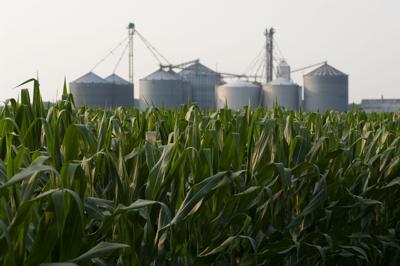The image displays a vibrant, close-up view of a lush cornfield with tall, green corn plants. Some of the leaves are standing upright while others are folded over or lying on the ground. Dominating the background is a collection of eight large, silver silos, each shaped like wide cylinders with pointed tops. These silos are interconnected by a network of wires and are flanked by two tall tower structures. The right-hand side of the image features a small farm building in the top corner. The entire scene is set against a backdrop of a gray, overcast sky, amplifying the contrast with the bright, well-maintained green foliage in the foreground. This tranquil yet industrious farm setting suggests a blend of agricultural activity and possible water or power management.